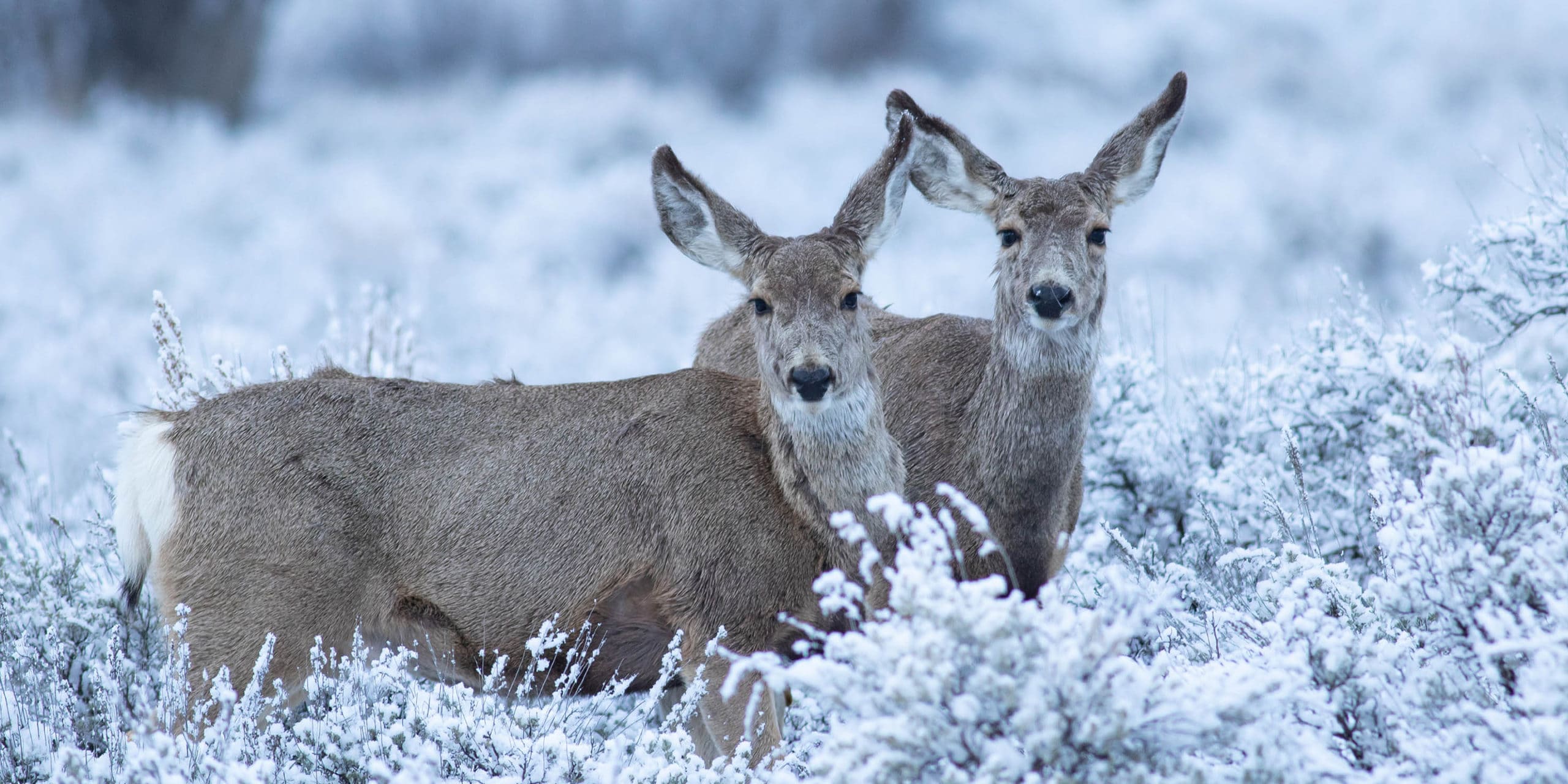In this detailed and evocative image, we see two deer standing close together in a snowy outdoor setting. The background is a wintry landscape, filled with trees and bushes heavily blanketed in a grayish-white snow, devoid of any greenery, with bits of black and white dotting the frost-covered foliage. Both deer, with their matted, brownish-gray fur, appear to be older and are exhibiting curious yet cautious expressions as they stare directly at the camera. Their black noses and eyes stand out starkly against the otherwise neutral and subdued color palette of the scene. The ears of the deer are particularly notable, showing a distinct white inner fur with black tips. One deer is positioned slightly to the middle left, turned directly toward the camera, while the other stands a bit behind on the right, turned partially to the side but still maintaining eye contact with the viewer. The surrounding environment is subdued and foggy, emphasizing the cold and stillness of the moment, and focusing the viewer's attention on the tan and white contrast of the deer against the monochromatic snowy backdrop.